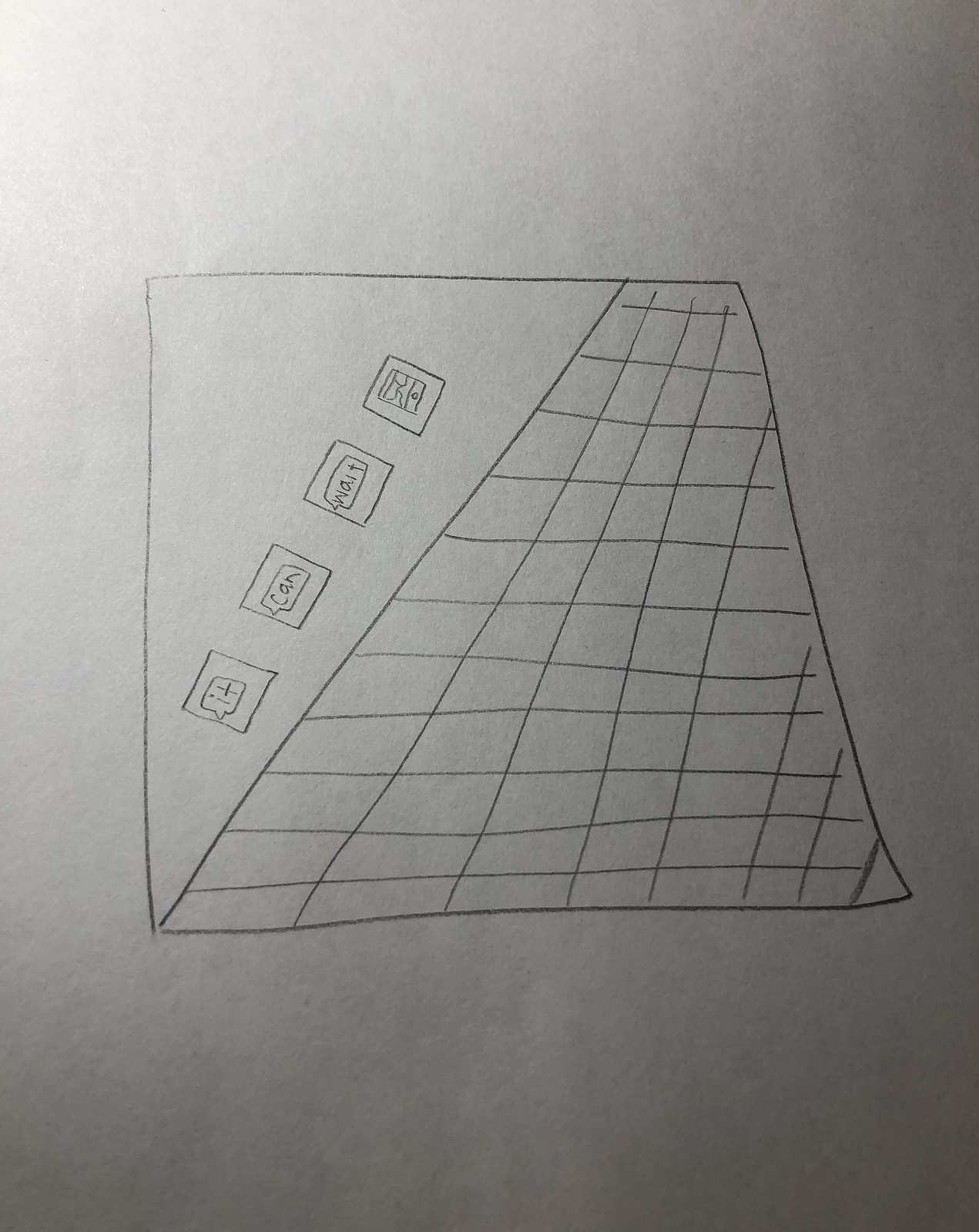The image showcases a drawing on a clean, pristine white sheet of paper. The light source, originating from the top left, casts dramatic shadows that darken the bottom right corner of the image while illuminating the top left corner, suggesting the light may be coming from an overhead lamp or natural sunlight. The drawing is executed solely in graphite pencil, presenting a monochromatic palette with varying shades of gray.

The sketch itself appears rudimentary and somewhat haphazard. The lines are uneven and disconnected in places, contributing to its overall unfinished and sloppy appearance. On the right side of the image, there's a checkered pattern formed by alternating squares. The pattern is part of a larger triangular shape, which slopes downward and narrows towards the right while widening towards the left. 

On the left side of the triangle, there are four smaller squares, each containing different elements. The first square from the left contains the word "it" encased in a bubble. Moving rightward, the next square has the word "can" in a similar bubble. The third square holds the word "weight" also in a bubble. The final square diverges from the text, featuring a rudimentary drawing of a map within its bubble.

Overall, the drawing is basic in composition and execution, characterized by its simplistic and uneven lines, with a distinct focus on geometric shapes and scattered text elements.